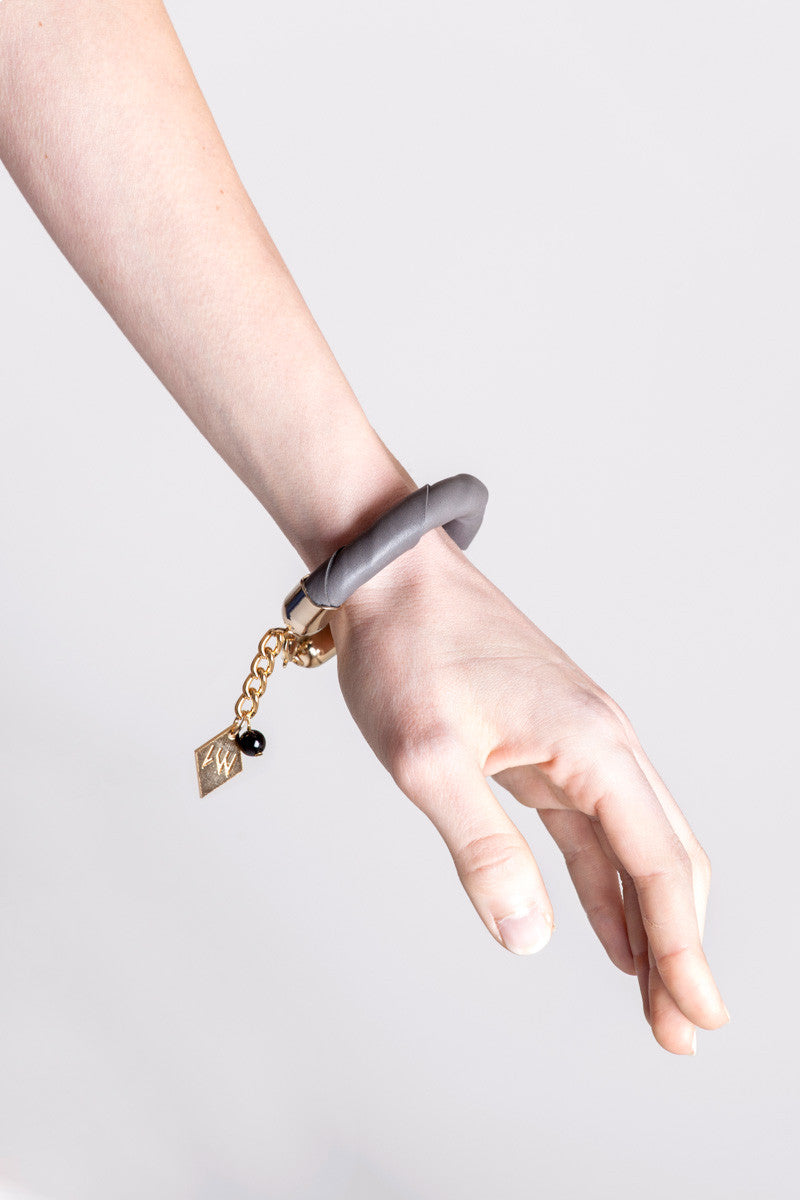The photograph depicts the left arm and hand of a pale-skinned Caucasian female, extending from just below the elbow to the fingertips, against a light gray background. On her wrist, a distinctive bracelet is prominently featured. This bracelet is wrapped in gray leather material and displays a gold segment where it clasps. Attached to this gold section is a delicate chain, from which hang two charms. One charm is a diamond-shaped piece inscribed with the initials "M1" or "LW," while the other is a small black bead, both of which dangle elegantly beneath the wrist.